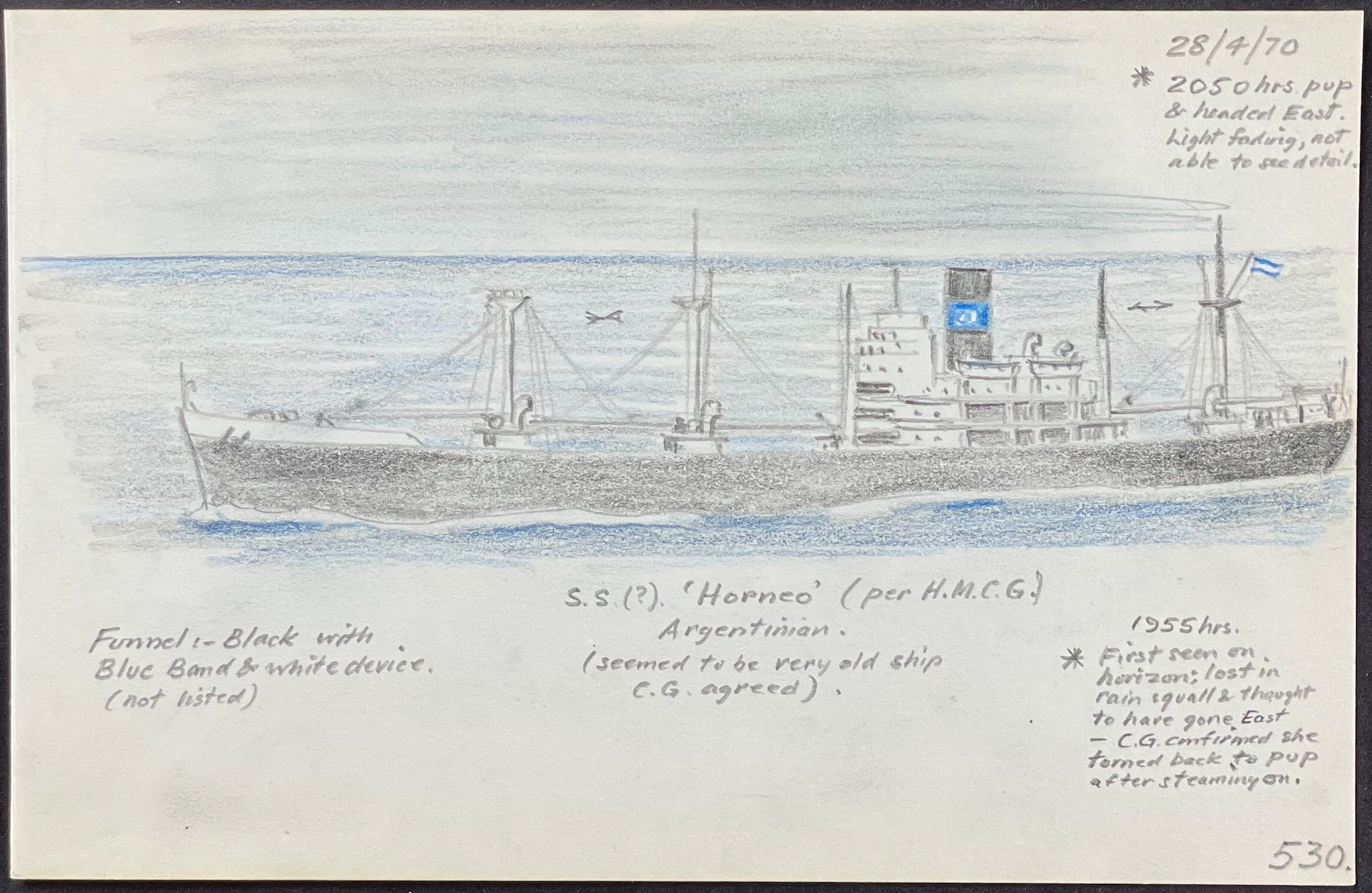This detailed illustration of a boat appears to be created using crayon or colored pencils, featuring shades of gray, blue, and white. Set against a water backdrop with a blue hue and highlighted by gray and white sky above, the boat itself is primarily black with white accents on the top and a distinctive white and blue flag. A prominent black smokestack with a blue band stands out, along with an exhaust pipe.

Inscribed at the top right of the image are the numbers "28/4/70" followed by "2,050 hours." Nearby, there are phrases like "top and land," "east," and "light," but the remaining text is unclear. Below the boat, there is a note mentioning a "funnel in black and white with blue band and white device," with additional text indicating uncertainty about the name: "question mark" followed by "Horneo" (H-O-R-N-E-O) and the abbreviation "HMCG." The note continues indicating "Argentinian," suggesting the boat is an old ship agreed upon by CG, possibly referring to the Coast Guard. Further details mention "1955 hours" and "first seen on the horizon, lost in rain squall, thought to have gone." 

At the bottom right of the illustration, the number "530" is prominently displayed. Adding a layer of intrigue to this depiction are terms like "PUP at 100 east," and "light fading, not able to see detail." Overall, the artwork evokes a sense of historical mystery and maritime legacy, capturing a seemingly ancient Argentinian vessel possibly dating back to CG's records around 1955 hours.